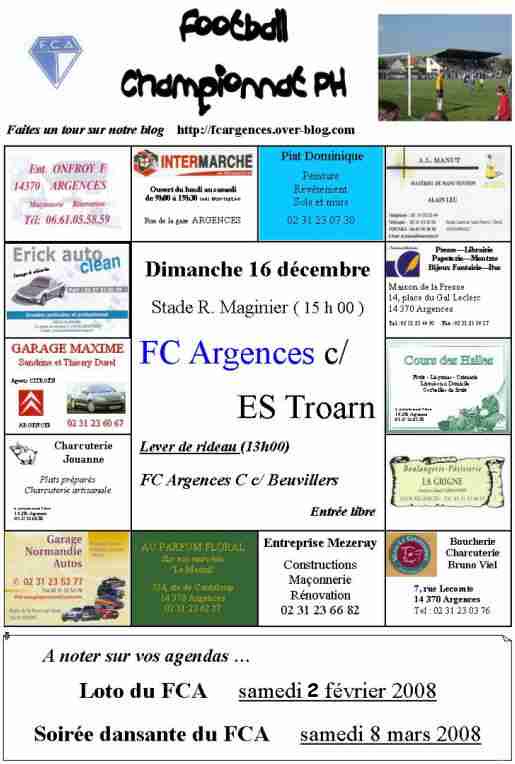The image is a detailed poster predominantly in another language, likely relating to a football (soccer) event. At the top left, it features a blue and white diamond emblem with the letters "FCA" in white. Next to the emblem is the phrase "Football Championship" in bold black letters. To the right of this text is a picture depicting a soccer field with a blue sky and green grass, where soccer players in yellow and red uniforms are in action.

Beneath these elements, there is a large box filled with multiple small advertisements arranged in a grid pattern—four along the top and several down the sides. In the center of this box, there’s a larger square containing key information in a mixture of languages, mostly non-English. It reads: "Dimanche 16 December, Stade Road, Meguineer, 15h00, FC Argences vs. C/ES Tron." This seems to be an announcement for a football match scheduled on Sunday, December 16.

Below the advertisement grid, there is a horizontal rectangular box with additional details about the event or organization, "FCA," along with some dates. The text here includes "fate un tour sur notre blog," which translates to "take a tour on our blog," and the URL "http://feargences.overblog.com." This part of the poster likely provides further information and points readers to an online resource for more details.